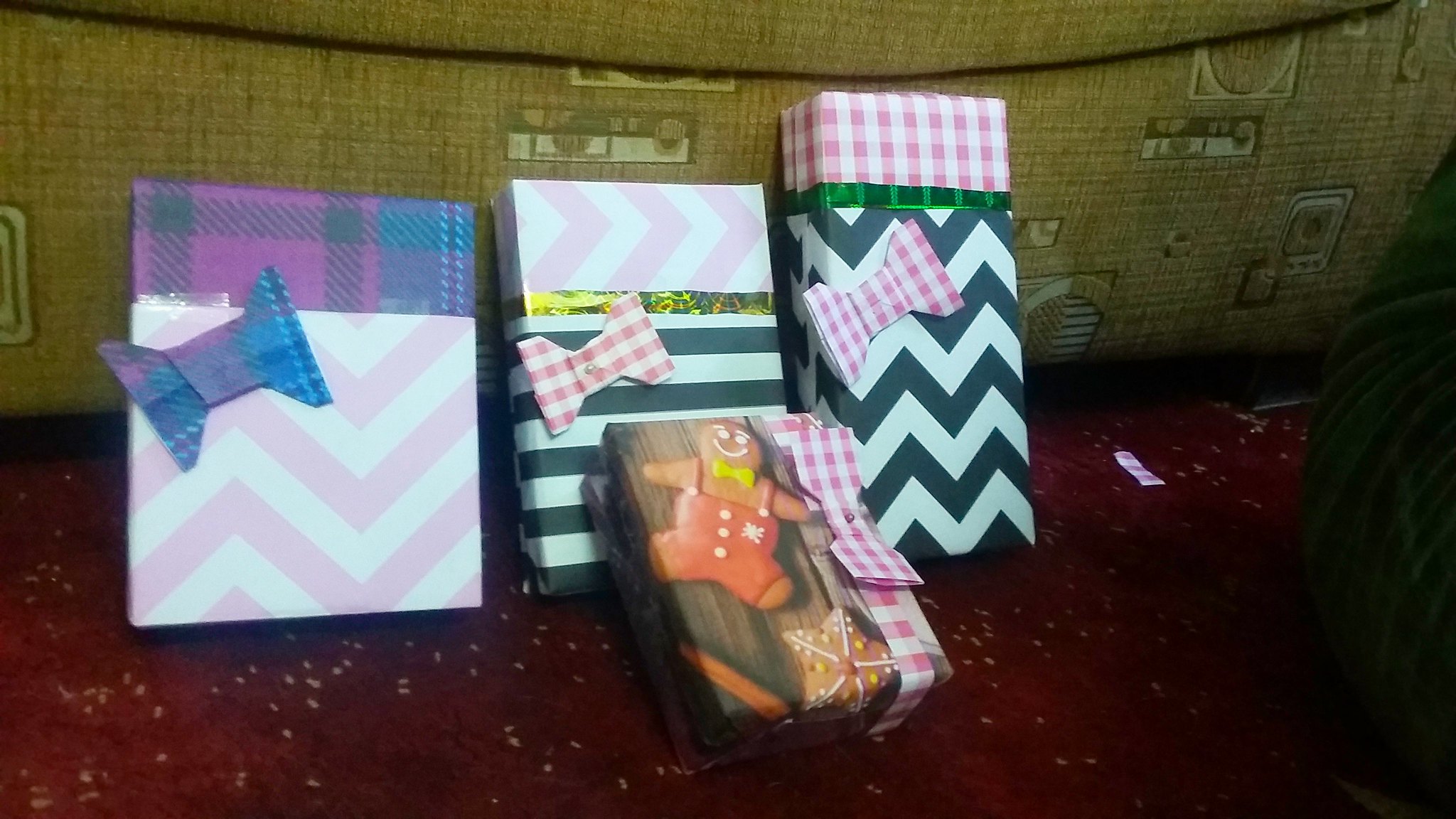This photograph depicts four presents arranged on a burgundy carpet, leaning against the front of a tan couch with a pattern of small brown squares. The presents, all different sizes and shapes, are wrapped in a variety of papers, showcasing a mix of plaid, zigzag, checkered, and thematic designs. 

The present on the far left features a top covered in purple and blue plaid, with the majority wrapped in white paper adorned with light pink diagonal stripes. A matching plaid bow sits on the left-middle corner. Next to it, a present combines wrapping papers: a quarter is pink zigzag on white, a quarter has green and gold accents, and the rest is white with dark green vertical stripes. It is finished with a small paper bow in pink and white checkers. 

In front of these, a smaller box resembles a shoebox, wrapped in paper that mimics wooden texture. On top, a gingerbread man decoration with white eyes, a white smile, a yellow bow tie, and brown suspender pants stands out. Below him lies another gingerbread figure with sprinkles, while a strip of pink and white checkered paper with a matching bow adds a playful touch to the presentation.

The final present in this arrangement has its top covered in pink and white checkers and is mostly wrapped in white paper with a dark green chevron pattern. This box also features a bow made of pink and white checkered paper. The setting is completed with specks scattered on the carpet, a piece of wrapping paper off to the right, and a glimpse of a floor plant beside the ensemble.